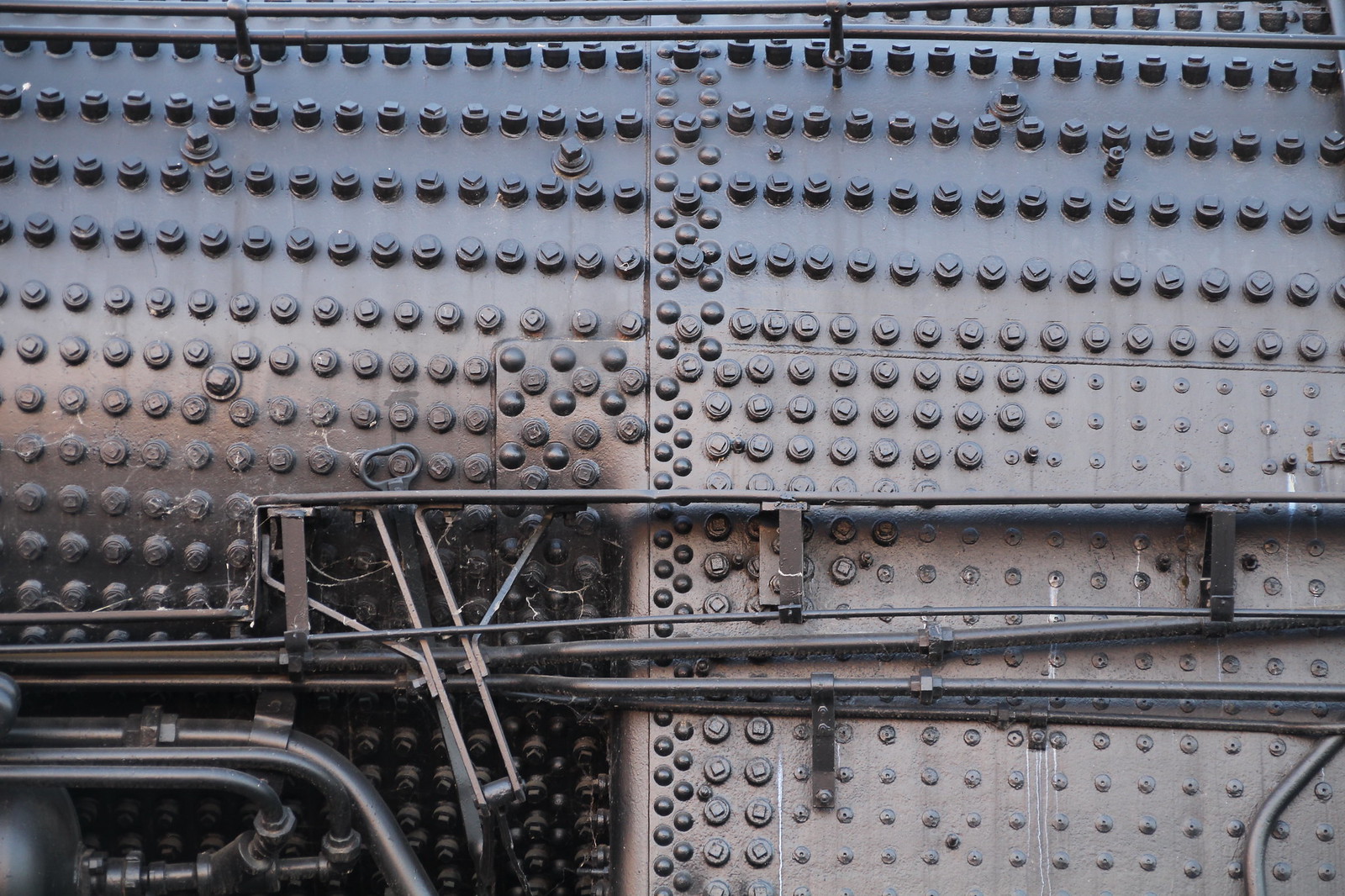The image depicts a large, industrial piece of equipment, resembling the exterior of a train engine or a similar mechanical structure. The surface is dominated by a vast expanse of silver-gray metal, densely studded with rows upon rows of circular bolts or rivets. Horizontal metal rods traverse the expanse, with a few situated near the top and around five more spanning the lower half. The bottom left corner features a cylindrical metal tank, reminiscent of a motorcycle tank, though clearly part of the industrial apparatus. This tank is connected to an array of black, cylindrical hoses that extend across and downward within the frame. The entire setup, with its intricate network of metal bars and pipes, suggests a highly complex and robust piece of industrial machinery.